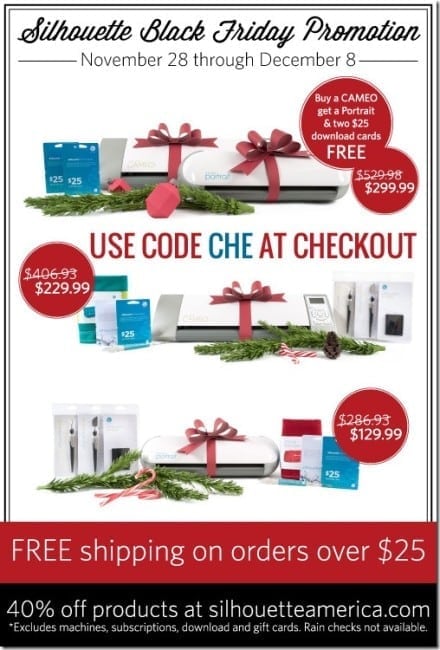The advertisement showcases a Black Friday promotion for Silhouette. In elegant cursive at the top, it reads "Silhouette Black Friday Promotion." Below this, the dates "November 28th through December 8th" are prominently displayed. Scattered throughout the advertisement are vibrant red bubbles with white text that highlight the offer details. 

One primary bubble states: "Buy a cameo, get a portrait and two $25 download cards free." The original price of $529.98 is visibly crossed out and replaced with $299.99. The ad also features images of the Silhouette Portrait device, $25 download cards, and a decorative green wreath. 

Additionally, a red text box directs customers to "Use code CHE at checkout," with "CHE" in bold blue. Adjacent to this, another red bubble shows a discounted price of $229.99, down from $406.93, for another bundle. 

On the right, a red bubble highlights a third product discount, reducing the price from $286.93 to $129.99, tied with festive ribbons. At the bottom of the ad, a red section announces "Free shipping on orders over $25," while a black section declares "40% off products at SilhouetteAmerica.com," with exclusions for machines, subscriptions, downloads, and gift cards. It also notes that rain checks are not available.